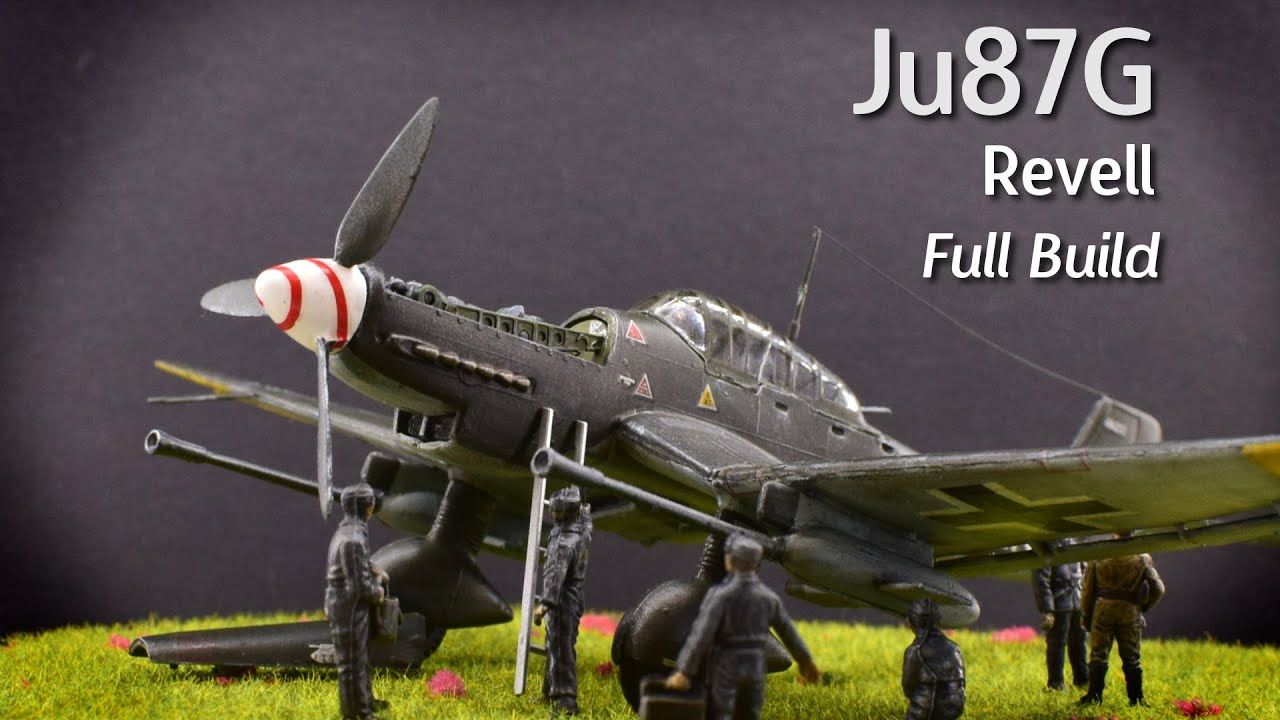This image showcases a detailed miniature model set featuring a military aircraft labeled "JU87G Revelle Full Build" in white font on the top right corner. The aircraft is predominantly dark gray with a distinctive white and red swirl nose, and a string extending from the top of the plane to its tail. Surrounding the plane are five figurines dressed in dark gray military uniforms, complete with long sleeves, long pants, and caps. These figures appear to be maintenance personnel attending to the aircraft. The scene is set on a field made of dark lime green grassy fiber material, with small pink bushes adding a touch of color to the predominantly green and gray palette. The background of the image is dark gray, enhancing the visual focus on the intricate details of the model set.